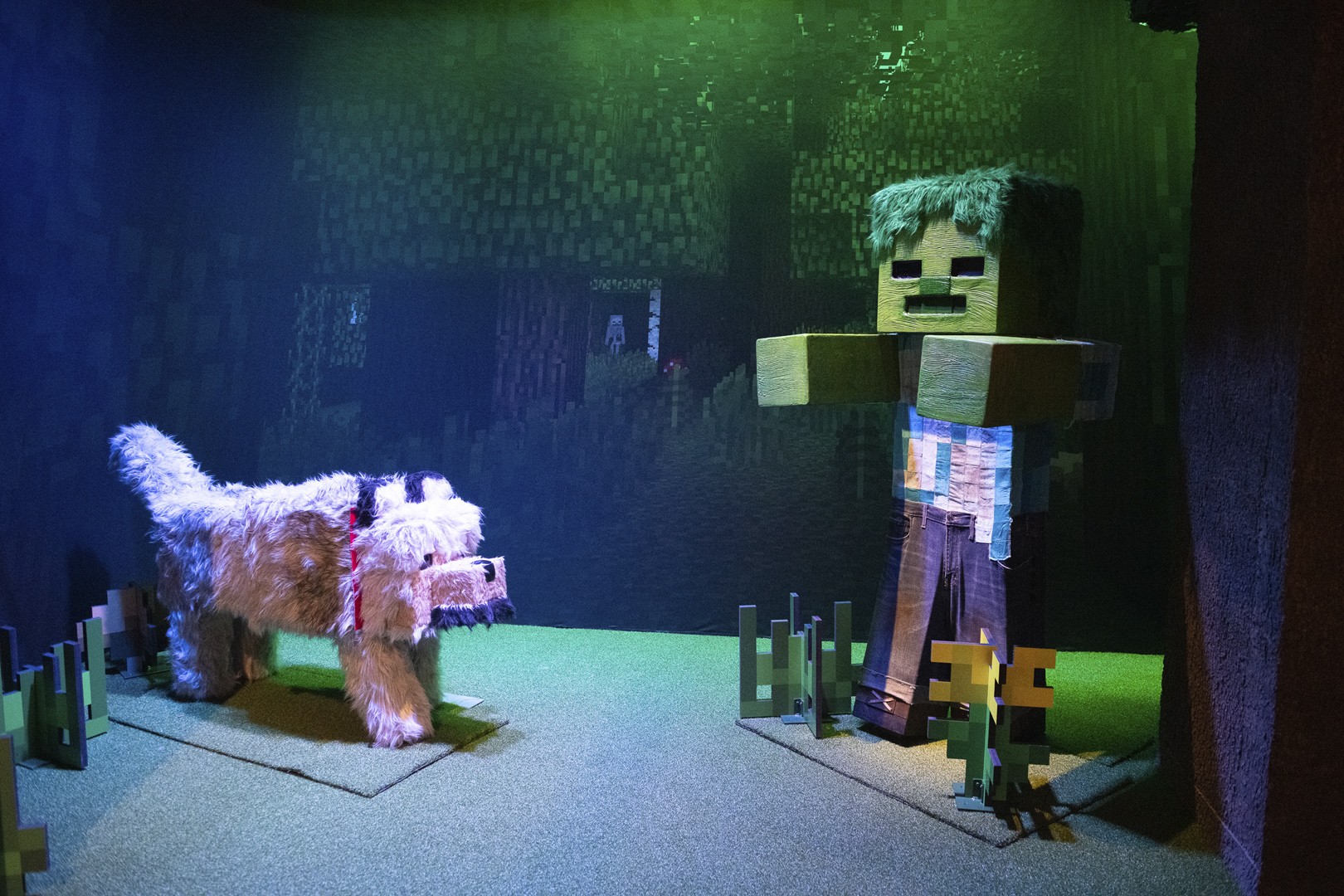This image depicts a vibrant Minecraft-themed art installation, vividly illuminated by green lights, which cast an emerald hue across the scene. On the left side, a dog, styled in Minecraft’s iconic blocky aesthetic, stands on a small gray rug. The pink dog, constructed perhaps from wooden boxes and fabric, features detailed elements resembling ears, a nose, and a collar. To the right, a formidable Minecraft zombie figure is showcased. This menacing character has a square head topped with what looks like green hair made from carpet, rectangular eyes, a gaping rectangular mouth, and outstretched rectangle arms. The zombie’s body, dressed in what appears to be paper mache clothing, stands atop pixelated wooden boxes. The background gives an impression of a man-made forest through the use of green hues, further enhanced by other box figures mimicking natural elements. The overall scene is meticulously crafted, with a combination of wood, cardboard, and fabric materials, creating a realistic yet fantastical diorama without any accompanying textual explanations.